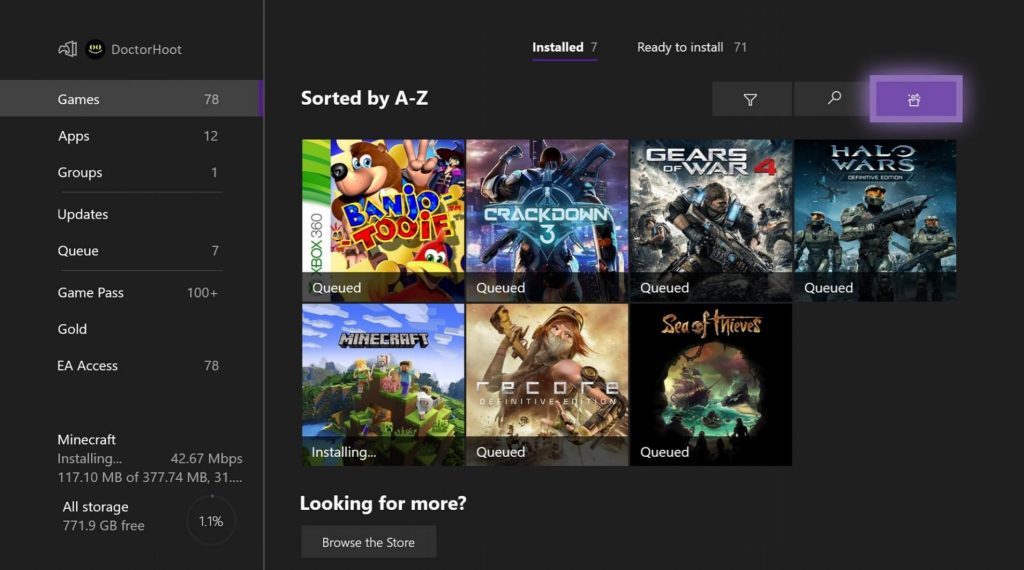The image features a user interface with a sleek black background. On the left side, a vertical menu is segmented by thin, horizontal lines. The first segment, highlighted in gray, begins with "Games" in white text, showing the number 78 beside it. Below this, "Apps" is bolded with the number 12, followed by "Groups" bolded with the number 1. Another line separates this section from the next, which lists "Updates," "Queue"—highlighted in this context—with a number 7 beside it.

Further down, divided by yet another line, appears "Game Pass" with the number 100, "Gold," and below that, "EA Access" showing 78. Continuing to the right side of the screen is a section captioned "Installed" (number 7), underlined by a vibrant purple line. Adjacent to this, it reads "Ready to Install" with the number 71, and "Sorted by A-Z" accompanied by an hourglass icon and a search button.

In the main section of the screen, seven video game icons are displayed in a grid: Banjo, 2D, Crackdown 3, Gears of War 4, Halo Wars, Minecraft, Rescope, and Sea of Thieves. Each game icon sits atop a semi-transparent black box labeled "Queued," except for Minecraft, which is marked as "Installing." At the bottom of the image, the text "Look for more" is prominently bolded in white, adjacent to a gray button with white text that reads "Browse the Store."